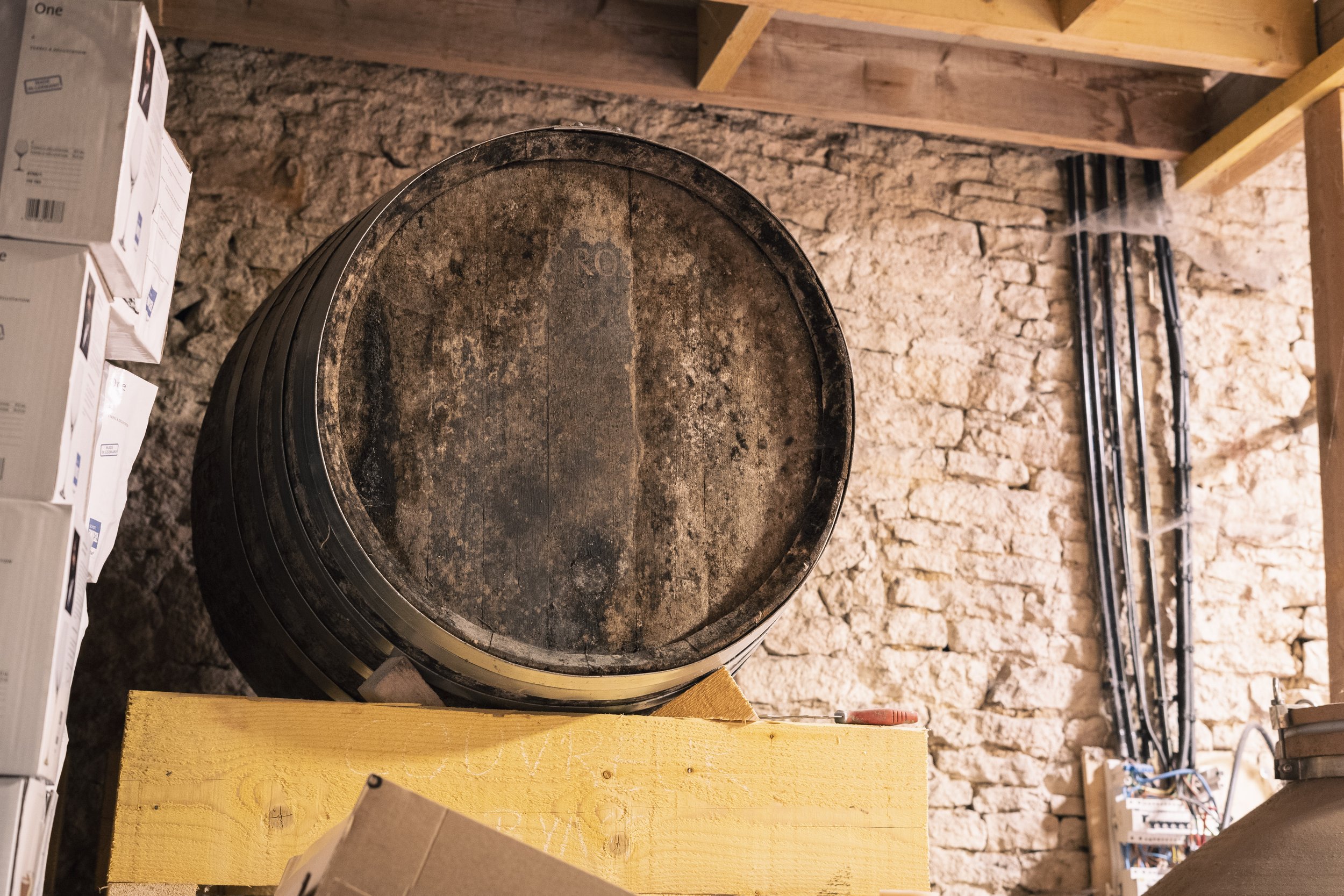The image depicts a rustic storage cellar featuring an aged wooden barrel prominently placed on a white wooden crate in the center. The background reveals a weathered, off-white, and slightly crumbled brick wall that exudes an aura of long-standing sturdiness. To the left of the barrel, a leaning stack of white boxes, some piled up high and slightly askew, adds to the cluttered atmosphere. The rough wooden beams of the ceiling suggest it may support stairs leading to an upper level. On the right-hand side, multiple electricity wires stream down the wall, indicating possible unfinished electrical work. The sunlight softly illuminates the room from the right, casting subtle reflections on the aged bricks. The entire setting gives an impression of an old, possibly under-renovation storage space, highlighted by the juxtaposition of rustic and modern elements.